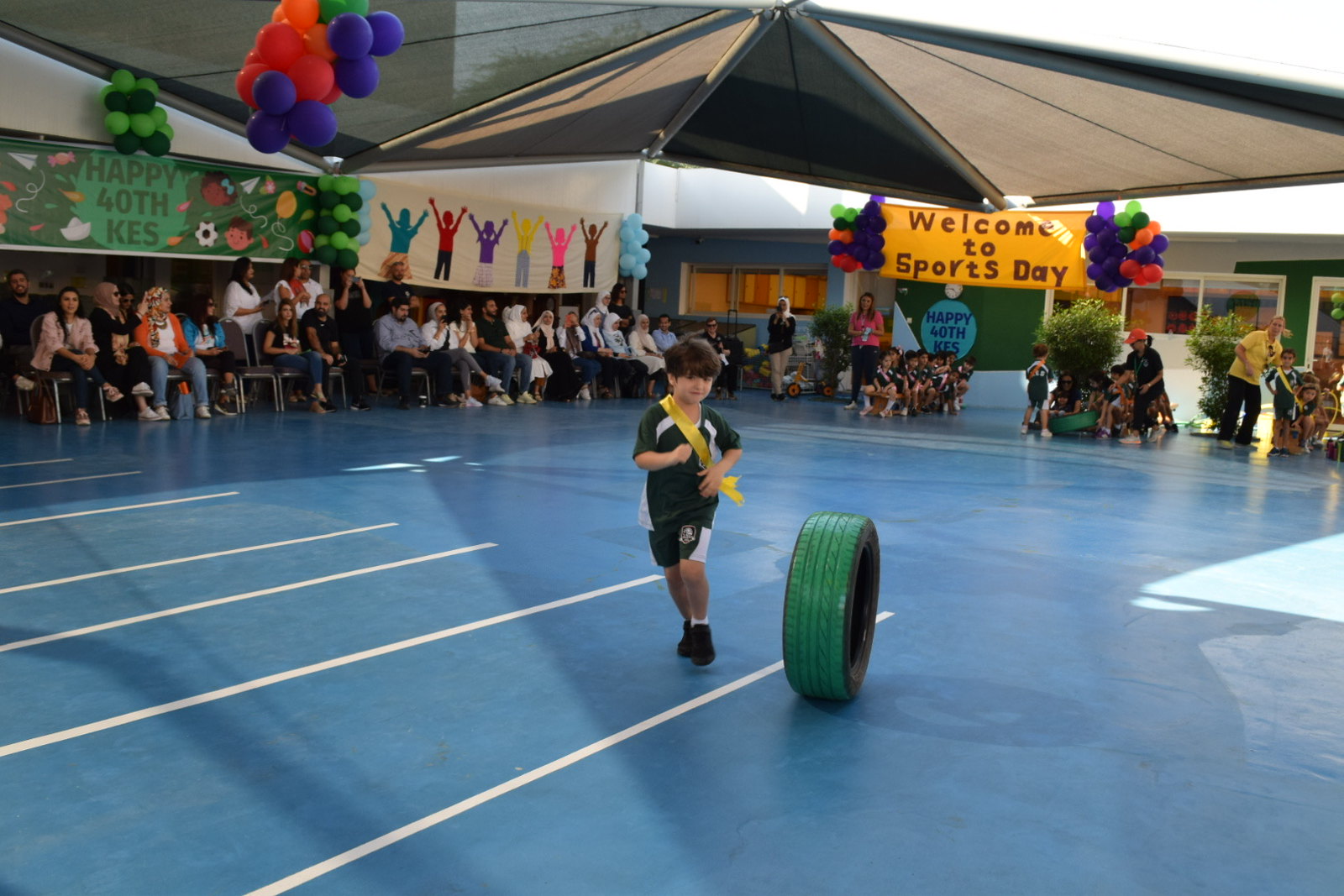In this vibrant image, a young boy is captured in mid-stride as he runs across a striking blue surface. He is dressed in a sporty ensemble consisting of black and white shorts paired with a matching black and white top, which gives the appearance of a jersey. Draped over his shoulder is a bright yellow sash that stands out vividly against his outfit. Beside him, an upright green tire adds an element of action to the scene.

In the background, a crowd of supportive adults can be seen watching the boy's energetic display. Above them, several colorful banners are strung up, adding to the festive atmosphere. On the left, a green banner reads "Happy 40th KES," commemorating the event. Adjacent to it is a white banner adorned with multicolored silhouettes of children joyfully raising their arms. Further to the right, a yellow banner welcomes everyone with the words "Welcome to Sports Day" written in bold red letters. Clusters of multicolored balloons are festively arranged around these banners, enhancing the celebratory mood of the event.